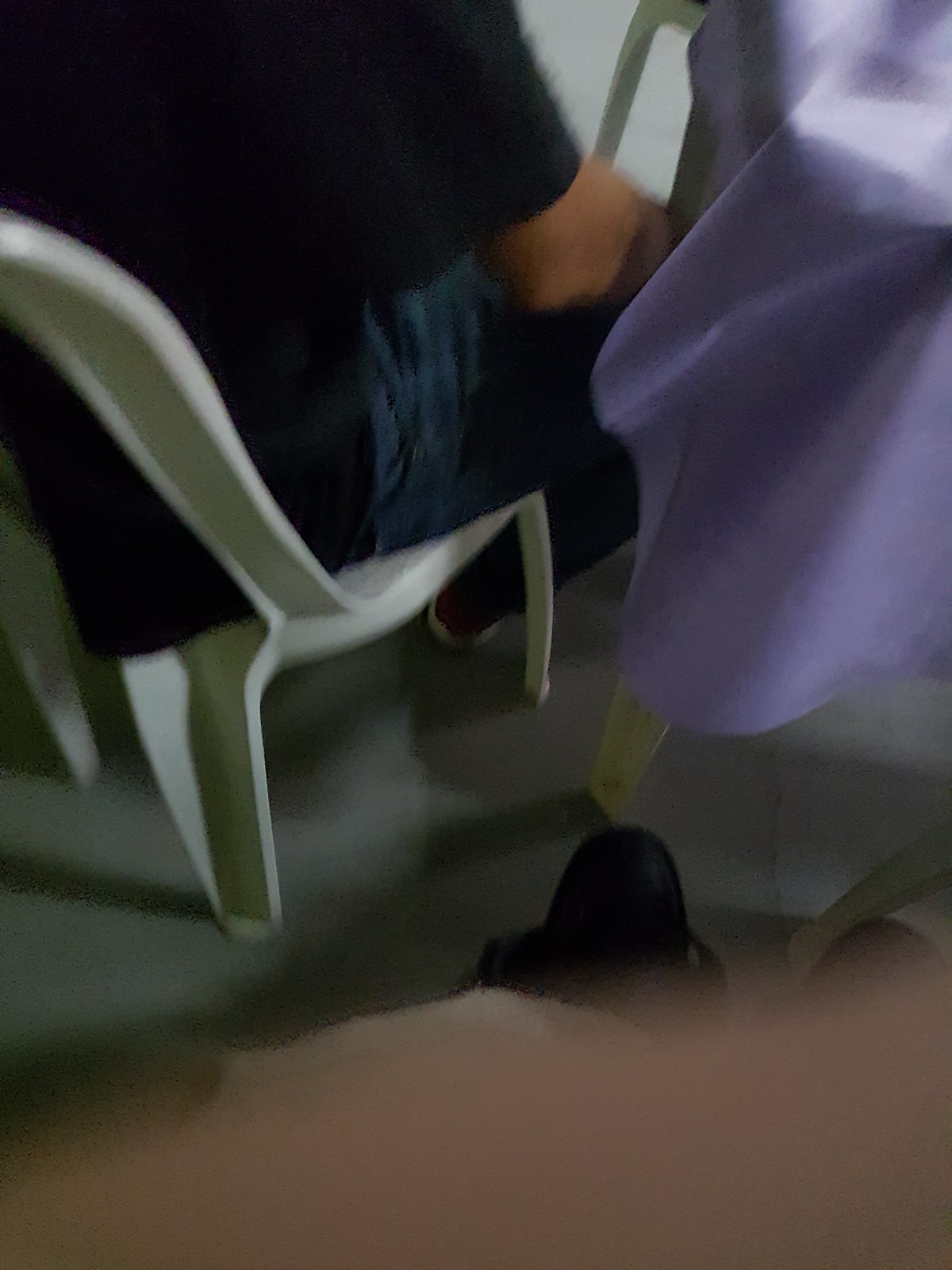A very blurry color photo depicts a medium-build, Caucasian man sitting in a cheap, white plastic chair, typically used outside on a deck. The image, taken from behind, reveals him wearing a black short-sleeve t-shirt, blue jeans, and shoes with white soles. The setting appears to be a makeshift dining area as he sits next to a matching white plastic table covered with a pink, satin-like tablecloth. The scene is shadowy and grainy, with part of the image obscured at the bottom, likely due to a finger over the lens. The gray flooring, possibly concrete or tiled, is flat and lacks texture. Scattered, indistinct objects are barely visible on the floor, adding to the overall blurry and unclear nature of the photograph.